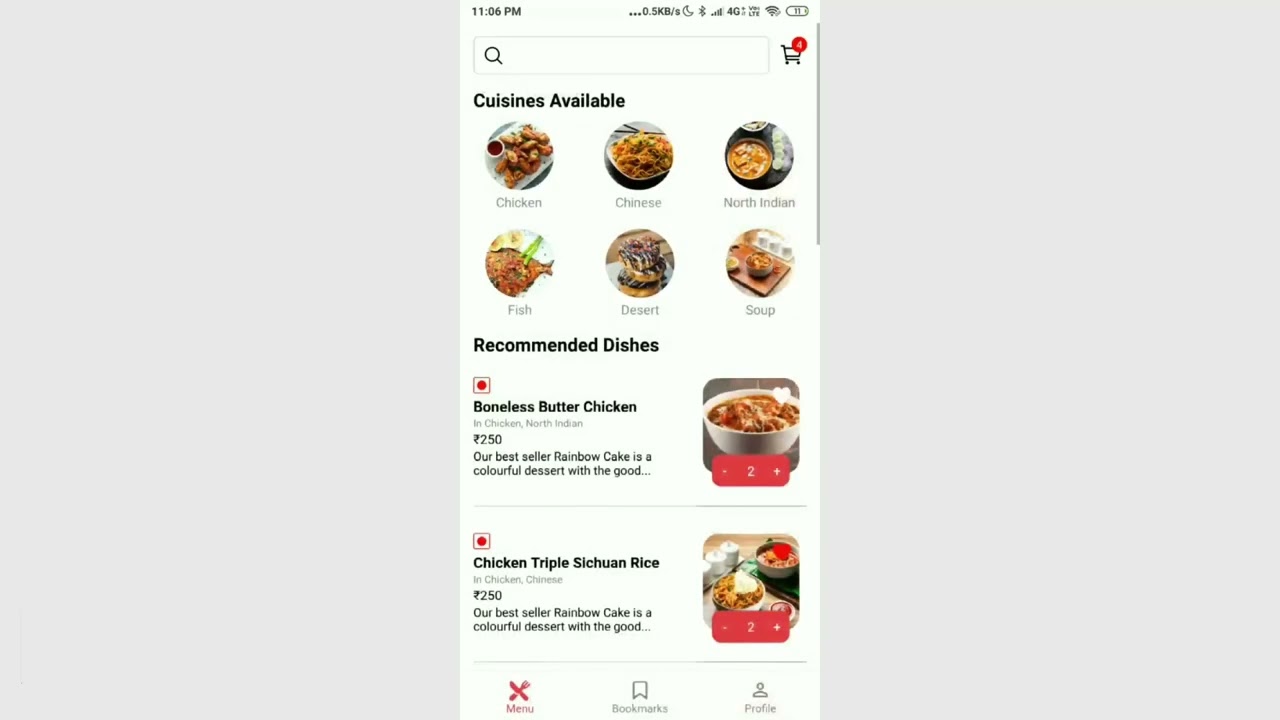**Screenshot Analysis of a Mobile Food Delivery App:**

The image captures a detailed screenshot from a user's mobile phone displaying a food delivery app. The interface is split into three sections with a prominent slim vertical rectangle in the center against a gray background. The time "11:06 p.m." is clearly visible in the top left corner, adjacent to the battery icon situated on the top right.

Below this, a search bar is prominently displayed, featuring a shopping cart icon on the right side. This icon includes a red notification circle indicating that items have been added to the cart.

The screen is divided into sections, with the first major section labeled "Cuisines Available." This area showcases a variety of dish categories each accompanied by an image:
- **Chicken**: Displayed with an image of cooked chicken pieces.
- **Chinese**: Illustrated with a picture of a plate containing Chinese food.
- **North Indian**: Represented by a bowl of traditional North Indian cuisine.
In the second row, there are categories for:
- **Fish**: Depicted with an image of a cooked fish.
- **Dessert**: Shown with a visual of cookie-like desserts.
- **Soup**: Accompanied by an image of a bowl of soup.

Further down, there’s a section titled "Recommended Dishes" in bold black text. Here, two dishes are highlighted:
1. **Boneless Butter Chicken**: Identified as "Our best seller."
2. **Rainbow Cake**: Described as "a colorful dessert with the good" (though the sentence appears to be cut off).

It is noted that the user has added two orders of Boneless Butter Chicken to the cart. Below this, another item, "Chicken Triple Szechuan Rice," is listed with two orders also added to the cart.

This comprehensive screenshot provides a clear view of the user's selected items and the diverse food options available within the app.